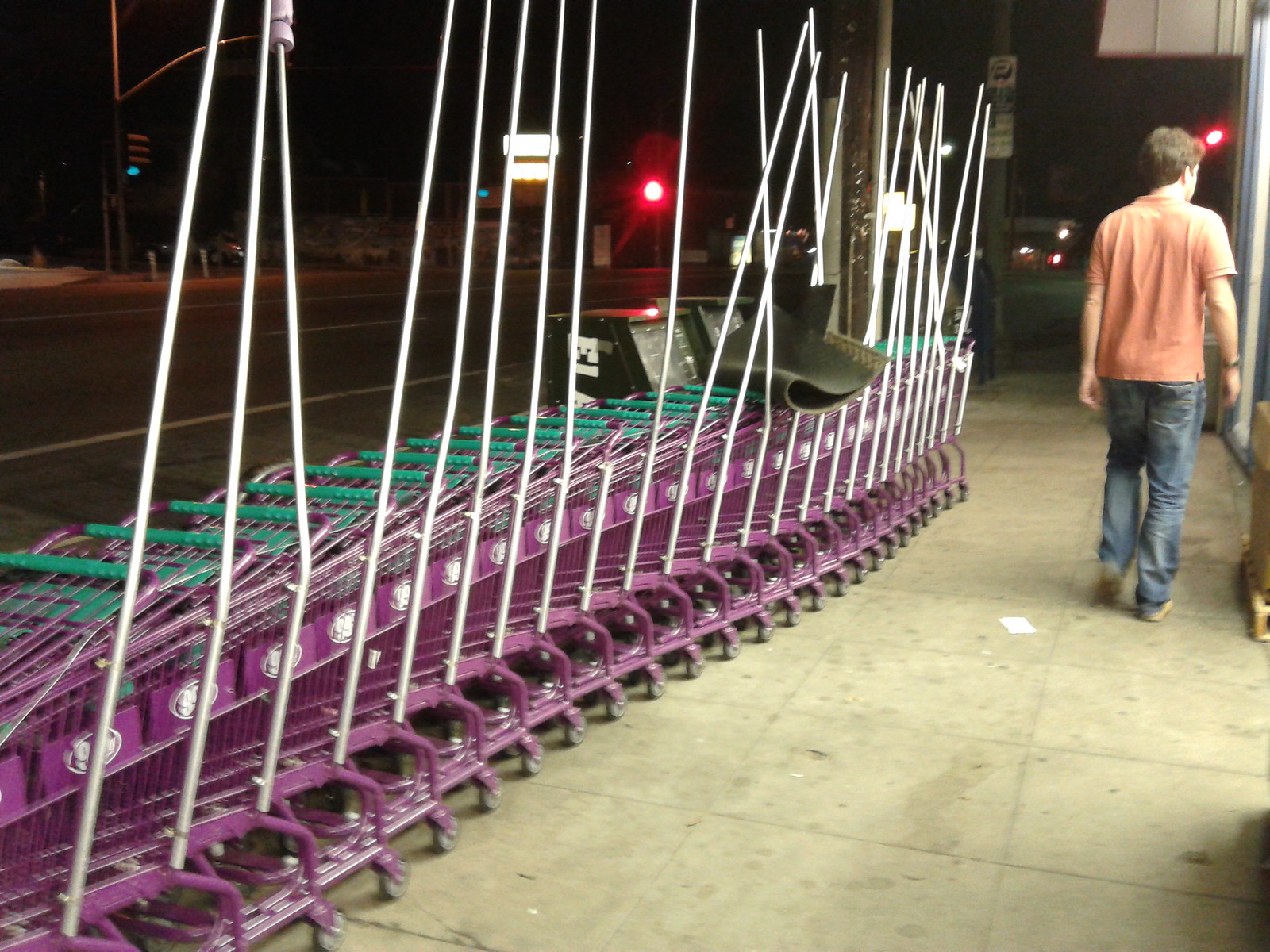In this nighttime photograph, a row of approximately 20-30 purple shopping carts with green handlebars sit outside in front of a store. Each cart has a long bar sticking up, designed to prevent them from being taken away. A doormat is casually thrown on top of one of the carts. Nearby, a man dressed in jeans and a short-sleeved apricot-colored shirt walks away on a dirty concrete tile sidewalk. In the background, two traffic lights illuminate the scene red, and a store sign is visible across the street. Newspaper boxes and stands are also positioned beside the carts.